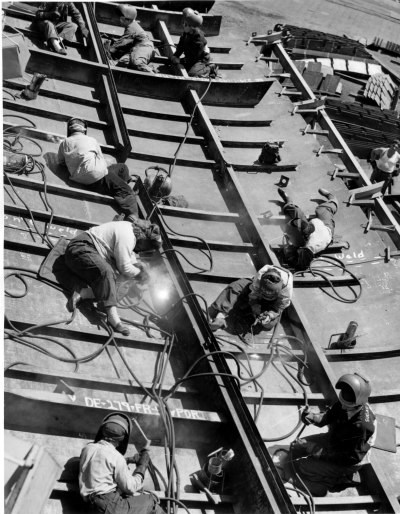This photorealistic, presumably old-fashioned illustration depicts a bustling construction scene with a significant focus on railroad assembly. At least eight men are meticulously working on the wooden ribs, which resemble the side hull of a ship, but appear to actually be part of a railroad structure. The workers, clad in white garb that includes elaborate headdresses, possibly white lab coat-style wraps, and wrist-length gloves reminiscent of dishwashing gloves, are laying on their sides, drilling amidst numerous spaghetti-like pipes and cords strewn around them. In the foreground, two men don welding masks as they operate their tools, connected by several cords. The black and white nature of the image, combined with the workers' old-fashioned attire and equipment, suggests that the scene dates back to a time when trains were a relatively new technology and a primary mode of transportation. The background reveals a more advanced stage of the construction effort, with some men having their welding masks lifted, working diligently under supervision. Additionally, a man in a dirty undershirt, possibly the manager, observes the progress, lending an air of oversight to the methodical and collaborative work environment. The overall scene is one of coordinated labor and technological development.